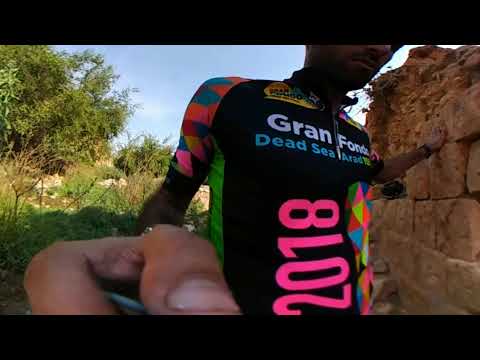This close-up photograph captures an African man from the middle of his nose down to his waist, highlighting his dark brown skin and a vibrant, tight-fitting shirt. The shirt, predominantly black, features an array of colorful geometric patterns, including pink, yellow, blue, orange, and black diamonds on the shoulders, with lime green sides. The most striking detail is the year "2018" in large, vertical, hot pink numerals. Horizontally across the chest, the shirt reads "Grand Fond Dead Sea Arad" in white and light blue text. His right hand, partially visible with the thumb in the foreground on the left, rests near a light brown brick wall on the right side of the photo. The background on the left showcases green grass and trees, adding a natural contrast to the vibrant attire.